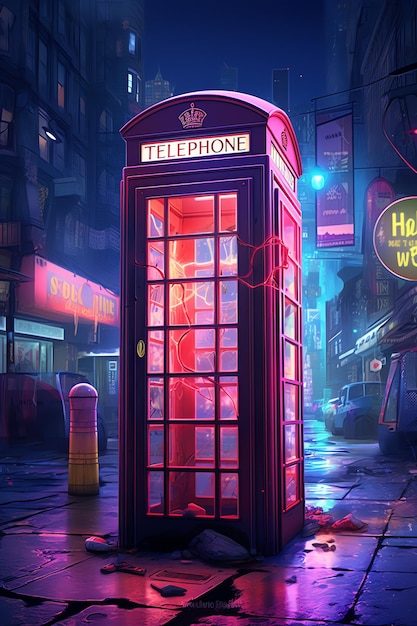This computer-generated photograph depicts a vibrantly colored, red and purple, European-style telephone booth with an otherworldly twist, prominently situated in a dark, deserted city street. The booth features clear glass panels on all four sides, bordered by sturdy beams in maroon or brown hues, and adorned with a lit sign labeled "TELEPHONE" in capital red letters on each side. Inside, glowing red and purple accents seem to pulsate like energy, while eerie, organic-looking red strings or veins stretch out, enhancing the magical ambiance. The booth's door handle is gold, adding a touch of classic elegance.

Surrounding the telephone booth are urban elements: to the left, a line of buildings with a noticeable neon sign in red, and a colorful safety cone transitioning from yellow to orange to pink. In front of one building, cyan lighting spills out, next to a green dumpster. On the right side of the scene, there are more buildings and a gray car that appears to be broken down. The damp, stone-paved street mirrors the glow of various neon lights, creating a surreal night-time atmosphere. The cityscape in the background features large buildings, suggesting the presence of restaurants or stores with their signs lit up in the night.

Overall, the scene radiates a mysterious, almost magical feel, reminiscent of a Doctor Who episode where the iconic character might have parked his time-traveling booth.